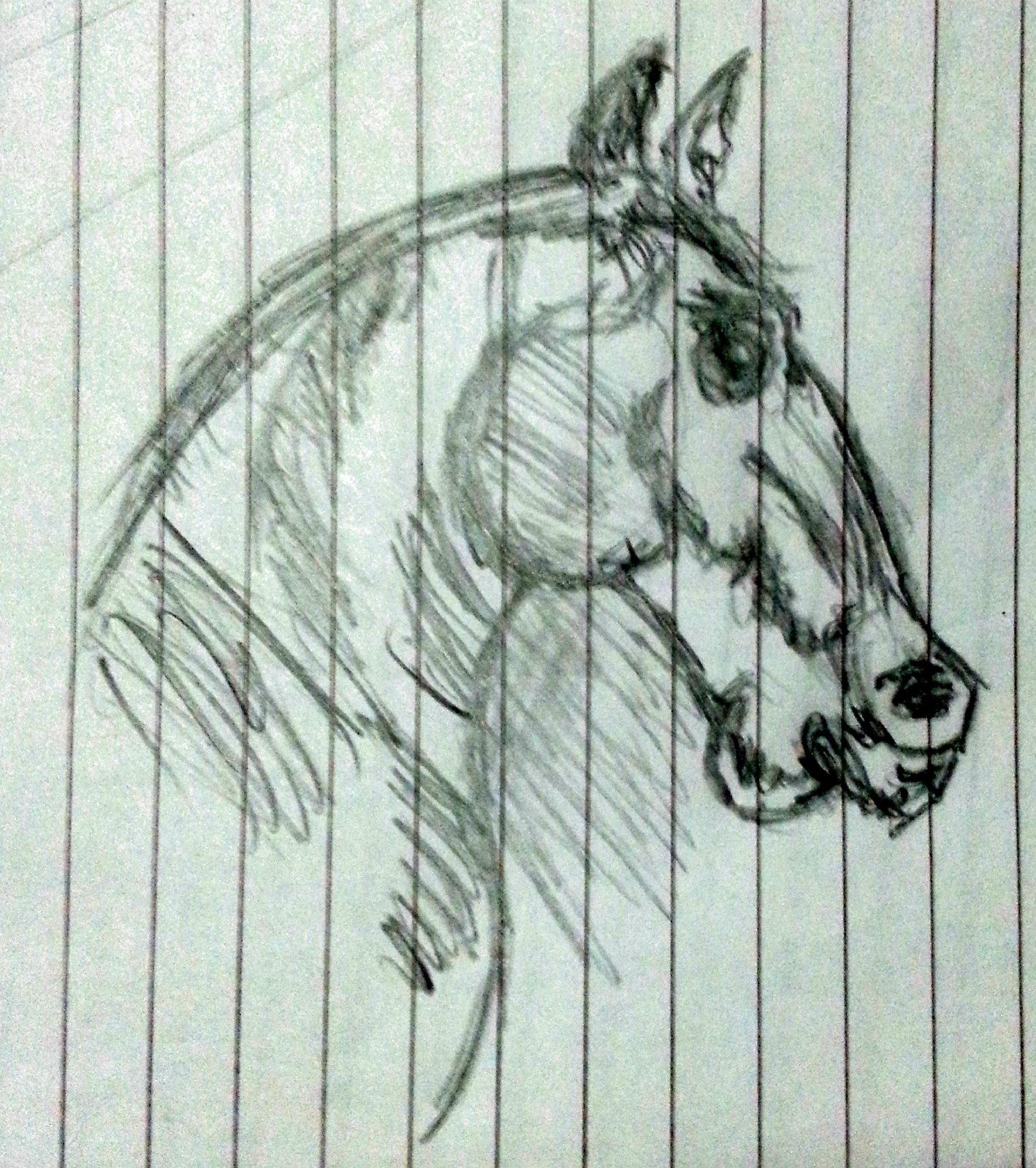On a vertically lined sketch pad resembling college-ruled paper, there is an intricately detailed pencil drawing capturing the profile of a horse's head and upper chest. The depiction showcases the horse's head, neck, and the beginning of its back with remarkable precision. The artist has meticulously illustrated features such as the horse's eye, cupped pointed ears, jawline, upper nose, and nostrils, even hinting at some visible teeth. The shading and shadowing masterfully highlight the curvature of the neck and the musculature of the front shoulders. Despite its scribbly appearance, the drawing exudes a delicate beauty and exceptional accuracy, bringing the horse to life on the lined paper.